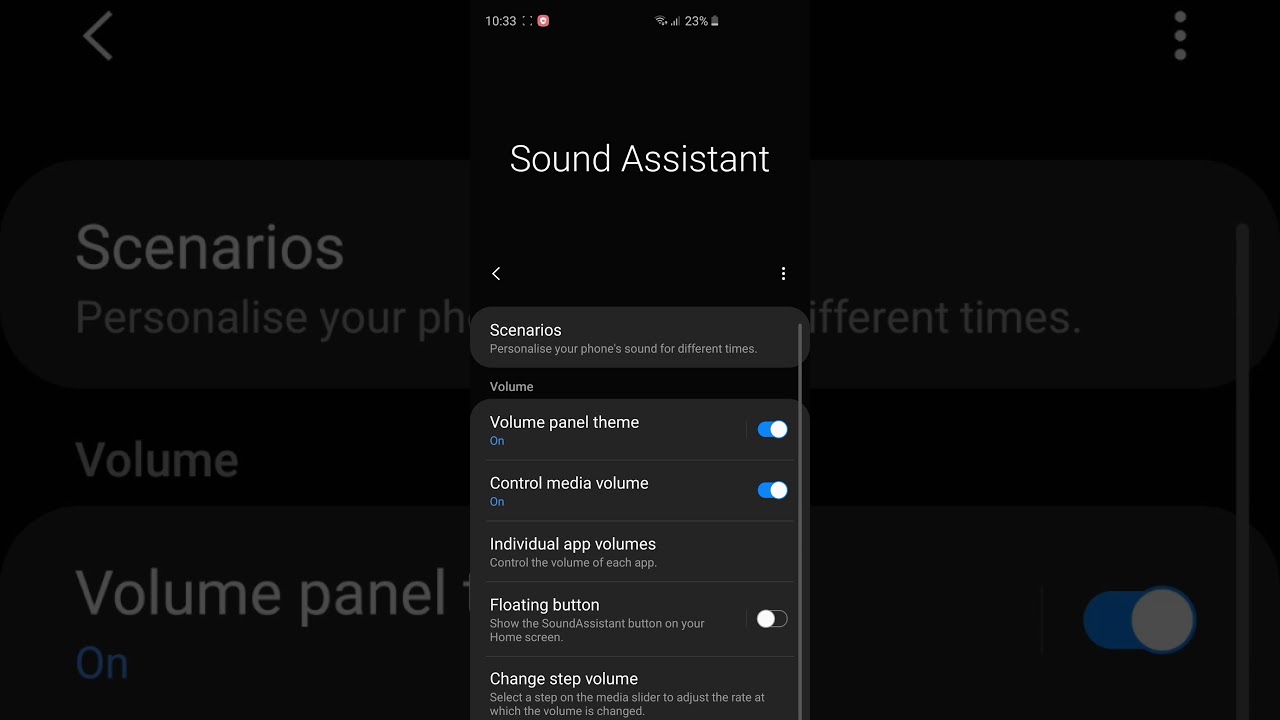A dark-themed preferences menu screen for a mobile app titled "Sound Assistant" is prominently displayed in the center of a nearly black screen. The vertical menu, centrally positioned, offers a variety of sound customization options. At the top, the menu begins with "Scenarios", which allows users to personalize their phone's sound settings for different times. Below this, there is a "Volume" section featuring several toggle options, including "Volume Panel Theme", "Control Media Volume", and "Floating Button". Another setting enables users to adjust the volume for individual apps and alter the "Change Step Volume". In the top right corner, a three-dot menu icon suggests more options or a pathway to a previous menu. At the very top of the screen, the current time and battery life of the device are displayed.